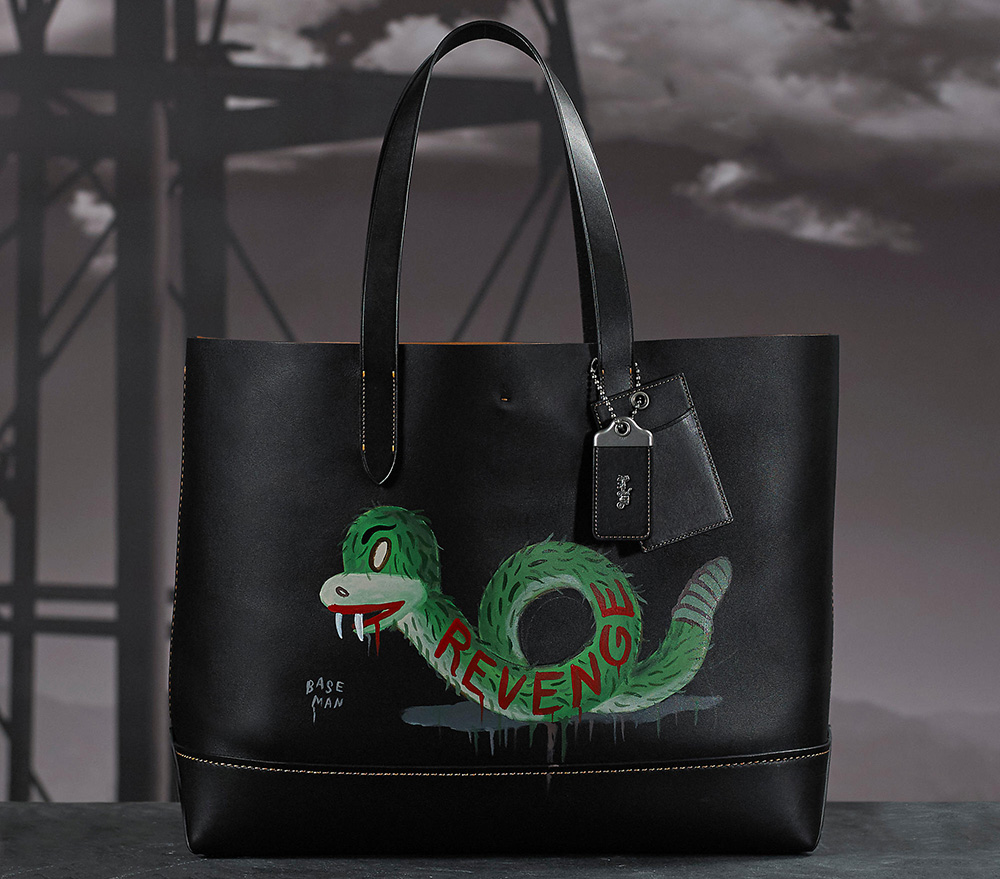The image showcases a sleek black leather handbag, positioned on a concrete ledge against a night sky with moody, dark clouds. The bag is adorned with intricate artwork featuring a green, slightly furry snake with white fangs and a somewhat rudimentary appearance. The snake has a white, pupil-less eye outlined in red, and a black eyebrow arched above. Its red lips drip blood, adding a dramatic flair. The word "REVENGE" is prominently written in red along the snake's body, and below it lies a white puddle. The bag also bears the text "BASEMAP" in capital letters. A black handle extends vertically from the top of the bag, accompanied by two black tags, one attached via a small silver chain. The background includes metal poles and a structure, contributing to the ominous atmosphere of the scene.